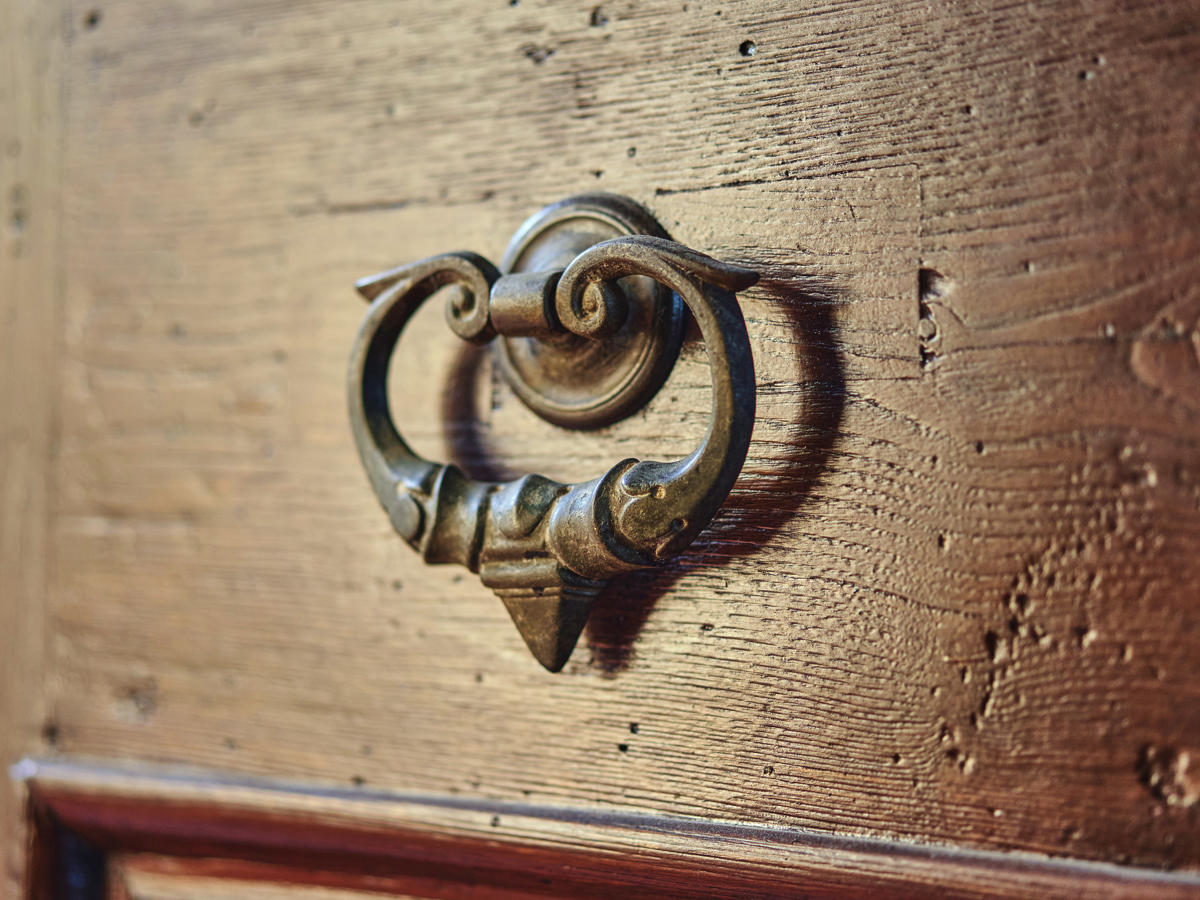This close-up photograph presents a detailed view of a brass metal handle attached to a reddish-tinted wooden surface, which could be part of either a door or a drawer. The handle, centered within the image but slightly facing to the left in a side view, features a round base flush against the wood, from which a small cylindrical piece extends outward. On either side of this cylinder, the handle curves upward, forming loops that curl back into the middle at the base. This terminates in a small pyramid-shaped piece pointing downward. Notably, the wood, which appears painted and possesses small dents and tiny potholes, runs from the left side of the image down to the bottom right corner, where a border possibly delineates one drawer from another. The photograph's focus highlights the right side of the handle, leaving the left side and some surrounding wood surface in a slight blur, further emphasizing the craftsmanship and detail of the metalwork against the aged wood.